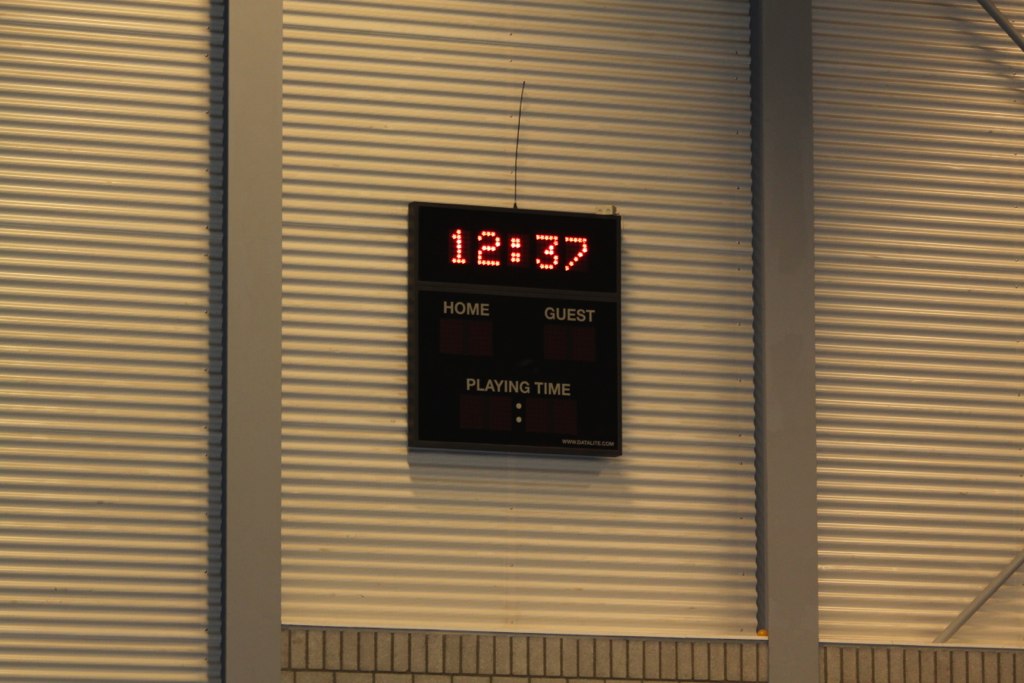This image captures an electronic scoreboard prominently displayed in a gymnasium. The scoreboard hangs on a wall covered with rippled metal paneling, providing a textured backdrop. The digital display shows the time as 12:37, though no game appears to be in progress as both the home and guest scores are blank. The absence of any indication of playing time further suggests that the scoreboard is not currently in use. A black electrical cord, or possibly an antenna, extends from the device, indicating its electronic nature and potential connectivity to a remote control system. The scene appears quiet and empty, focusing solely on the dormant scoreboard awaiting its next activation.